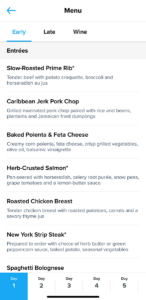A slightly blurry screenshot of a phone screen displaying a restaurant menu. At the top of the screen, a blue back arrow is positioned to the left of a banner labeled "Menu." Below the banner, there are three headings: "Early," "Late," and "Wine," with "Early" highlighted in light blue and underlined, while "Late" and "Wine" remain in black. This suggests different menu categories. Underneath, the heading "Entrees" is followed by a list of dishes, each with a brief, hard-to-read description in gray text. The entrees listed are:

1. Slow Roasted Prime Rib
2. Caribbean Jerk Pork Chop
3. Baked Polenta and Feta Cheese
4. Herb Crusted Salmon
5. Roasted Chicken Breasts
6. New York Strip
7. Spaghetti Bolognese

At the bottom of the screen is a banner divided into five squares, each labeled "Day 1" through "Day 5," presumably indicating different menu options for each day. The screenshot captures someone navigating this menu on their phone, likely preparing to order food.